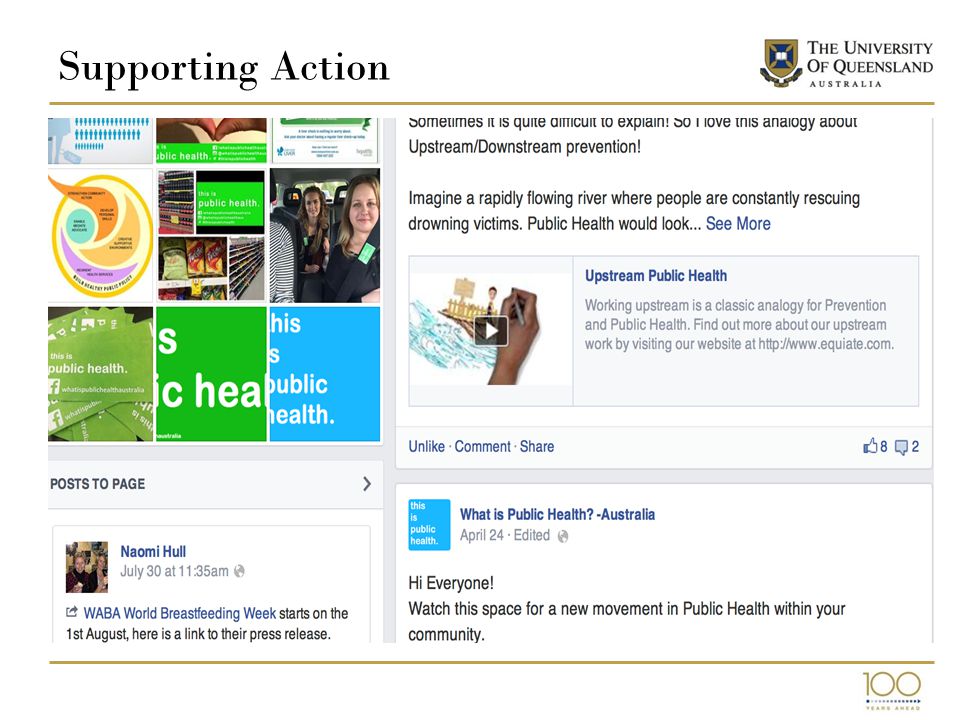Here's a detailed and cleaned-up caption for the described image:

---

This screenshot is of a website associated with the University of Queensland, Australia. The website features a banner at the top left reading "Supporting Action." On the top right, the name "The University of Queensland Australia" is displayed alongside the university's logo. Below this header is a gold horizontal line dividing the page.

The main section of the screenshot showcases what appears to be embedded content from a Facebook page. In the top left corner of this section, there are thumbnails of various posts made by the page. On the top right, there is a highlighted post that begins with the words, "Sometimes it is quite difficult to explain so I love this analogy about upstream and downstream prevention. Imagine a rapidly flowing river where people are constantly rescuing drowning victims. Public health would look..." followed by a "See More" option, which is highlighted in blue.

Beneath this excerpt, there is a link to a video, with interactive options to like, comment, or share the post. Additionally, the post shows it has received 8 likes and 2 comments, indicated by the thumbs-up icon and comment bubble, respectively.

Another post is visible just below. Titled "What is Public Health Australia," it is dated April 24th and marked as edited. The post reads, "Hi everyone, watch this space for a new movement in public health within your community." Toward the bottom right of the screenshot, there is a number "100" followed by some smaller text that is not legible.

---

This detailed caption captures all visible elements and context of the screenshot, providing a clear and descriptive overview.